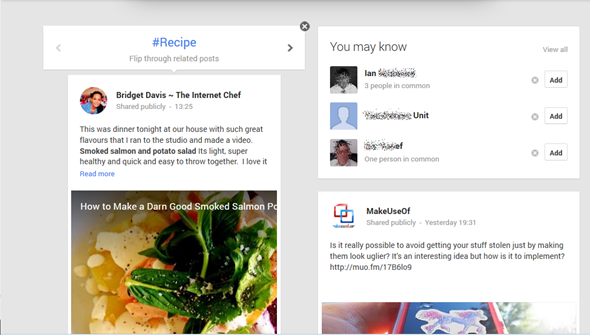"A vibrant culinary creation by Bridget Davis, the internet chef, showcases a plate of golden tortilla chips, artfully adorned with a fresh, green leaf garnish. Amidst various related posts, Bridget's recipe stands out, inviting food enthusiasts to delve into her flavorful dishes. Explore more of her tantalizing meals and culinary tips by flipping through her related content."